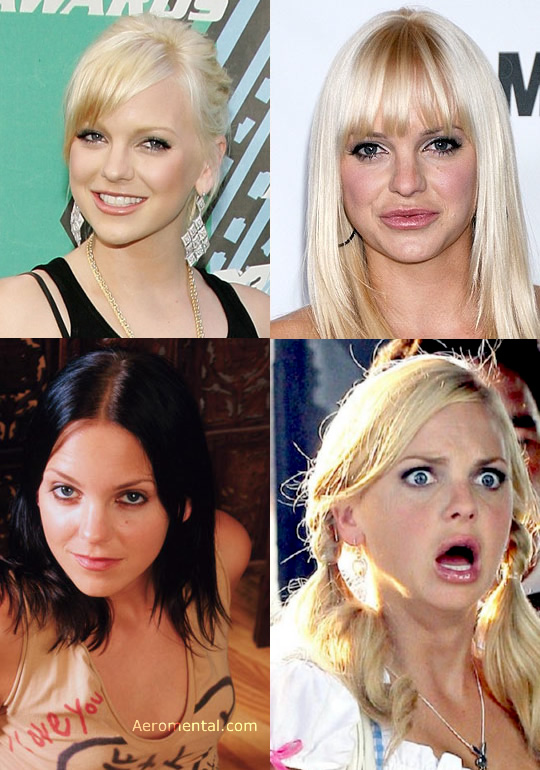The image is a large rectangle divided into four distinct headshots, likely depicting the same woman at different stages of her life. Each photo captures her with varying hairstyles, outfits, and makeup looks. In the upper left corner, a young, light-blonde woman with pale skin and diamond earrings beams a friendly grin directly at the camera, exuding an innocent, fresh-faced charm. The upper right photo features a similar-looking woman, now with bangs and a more glamorous, heavily made-up Hollywood appearance. The bottom left corner showcases a brunette with a "girl next door" vibe, characterized by her black hair and simple, down-to-earth look, yet still engaging directly with the viewer. The bottom right image presents a dramatic transformation with the woman sporting pigtails, plump lips suggestive of Botox, and an overall Hollywood-altered aesthetic. The background colors range from teal to light blue, with some gold and red elements, particularly in the lipstick colors. Visible but unreadable text appears in the top two photos, and there is some indistinct text at the bottom of the image as well. The women are all the focal point of their respective photos, each looking either directly at the camera or slightly to the side, with the context of the backgrounds remaining ambiguous.